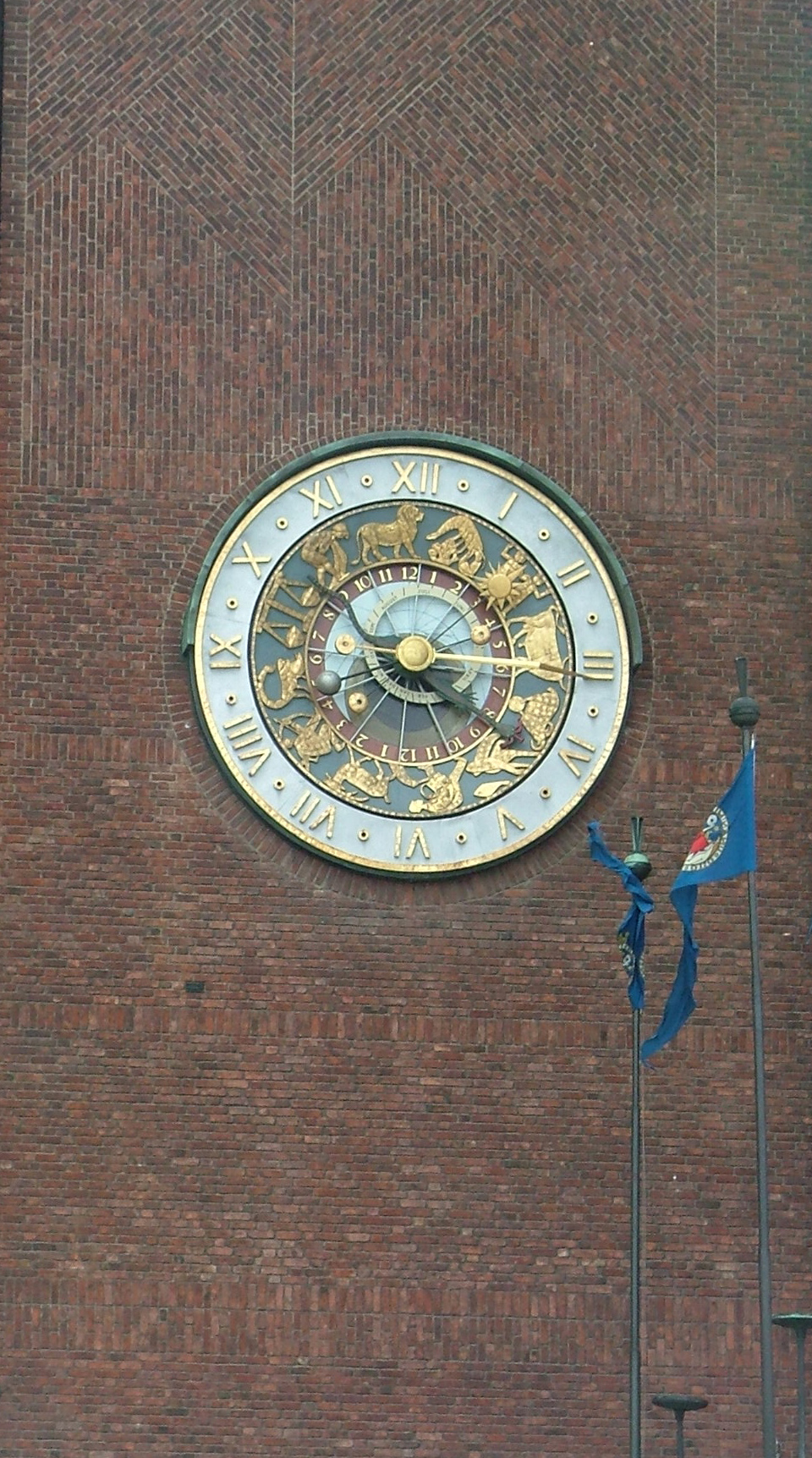The image showcases a prominent clock mounted on the red-brick exterior wall of an official-looking building, possibly a courthouse. The clock, likely positioned not too high up the wall, is flanked by two flagpoles bearing blue flags. The clock itself features an intricate design with Roman numerals on its outermost ring, interspersed with small dots. Encircling the inner section of the clock are gold symbols representing various astrological signs, such as a lion, scales, a crab, and a scorpion. Within this astrological circle, another layer features regular numbers in gold on a white banner, possibly for easier readability. Further inside, there is an additional rotating circle with visible turning mechanisms, indicating the time with its hands. The clock hands appear to be pointing to around 4:15. The rich colors of the clock and brick wall—blue, green, gold, red, white, and orange—combine to create a visually striking and detailed composition.